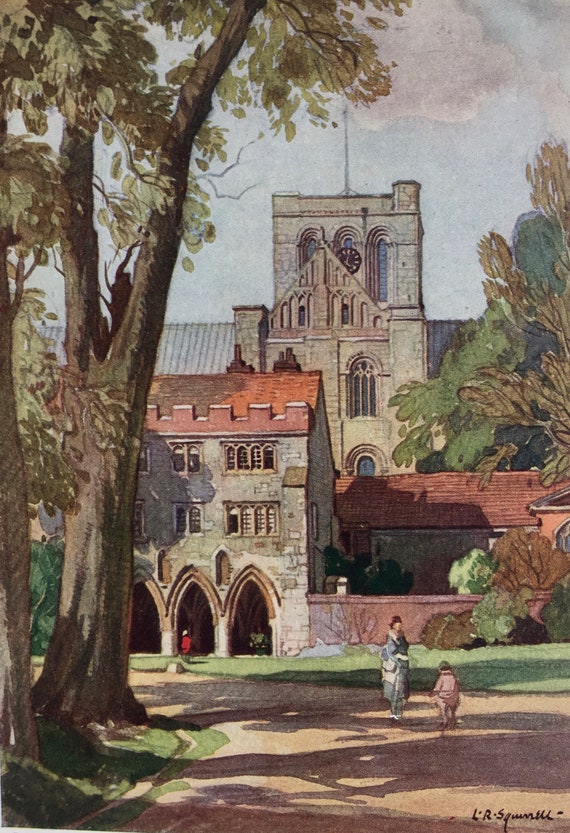This is a vertical rectangular painting, likely done in watercolors, showcasing a predominantly muted and softly colored depiction of a large, architecturally ornate building that could be an old school, monastery, or church, with a touch of characteristic features such as arched windows and entryways, clock tower, and intricate brick and stone details. The building is surrounded by trees, particularly to the left where there are some tall deciduous trees adjacent to a curved dirt-colored pathway. 

In the foreground, there are two figures - a woman in a blue dress or jacket, reminiscent of 1920s fashion, and a child in a tan or possibly pinkish outfit. Additionally, under one of the arched entrances, there is a person dressed in a striking red sweater or jacket, adding a vivid contrast to the otherwise subdued color palette. The roof tiles of the building are red, contributing a faint hue juxtaposed against the gray stone of the structure. 

The sky is bright blue, indicative of daytime, casting a serene yet lively atmosphere over the scene. The painting is signed in the bottom right, though the signature appears partially legible, potentially reading "LR” followed by a surname starting with an “S". The overall style strikes a balance between realism and abstraction, maintaining consistent perspectives and proportions without diving into intricate details.